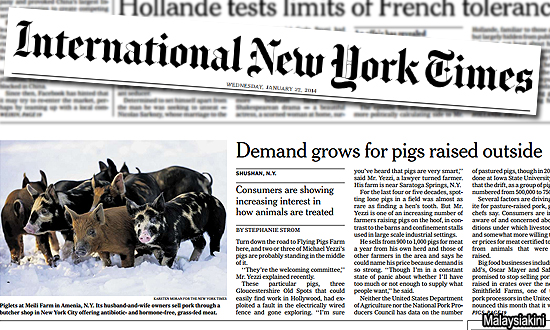A screenshot of a newspaper featuring two articles. The first article is titled "Holland Tests Limits of French Tolerance" and the second is "Demand Grows for Pigs Raised Outside." The latter discusses the increasing consumer interest in the ethical treatment of animals. Accompanying the articles is an image depicting a snowy scene with approximately five or six pigs. The caption for the image, written by Stephanie Strom, reads: "Turn down the road to Flying Pigs Farm here, and two or three of Michael Yeezy's pigs are probably standing in the middle of it. They're the 'welcoming committee,' Mr. Yeezy explained recently." The screenshot also includes a white rectangle with the text "International New York Times, Wednesday, January 27, 2014" in black.